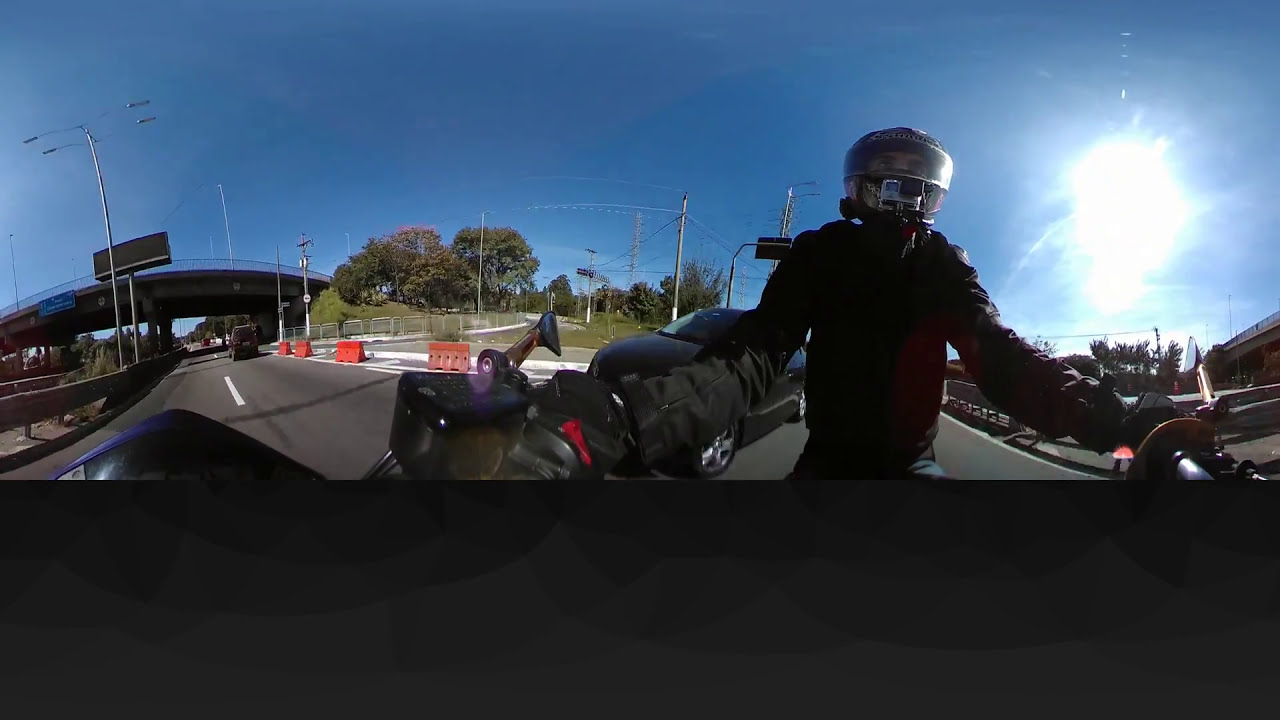A daytime selfie captures a motorcyclist, visible from the waist up, waiting in traffic on a black motorcycle. The rider is equipped with a black padded jacket, black gloves, and a black helmet with a clear visor pulled down. A gray and black GoPro camera is mounted at mouth level on the helmet. Both hands grip the motorcycle’s handlebars, which are positioned on a black asphalt road marked by a white dotted line indicating lanes. To the left of the rider, a black two-door car is visible in the adjacent lane. The sky above showcases a dark blue hue with the sun shining brightly, contributing to shadows especially around the rider's upper body. In the background, a cement bridge and some street lights are faintly visible. Electrical wires stretch across the skyline, adding to the urban landscape. The overall lighting and shadows confirm the picture was taken during daylight hours, with the sun positioned behind the motorcyclist.